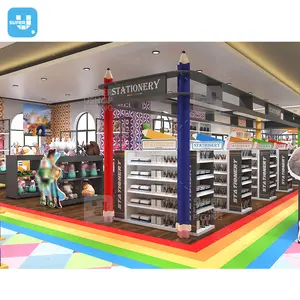This image showcases a vibrant stationery display within a store, distinctly marked by large rainbow-colored lines that segregate this section from the rest of the store. The centerpiece features two colossal pencils, each towering at approximately 10 to 12 feet high, with one being red and the other bluish-purple, serving as posts for the display. Nestled between these giant pencils is a gray banner that reads "STATIONERY" in bold white letters.

The display area contains racks shaped like diagonal pencils with colors including yellow, blue, orange, green, and red, each designated for different types of stationery products. There are four clearly labeled stations within this section. Adjacent to the stationery section, on the left, are two shelves filled predominantly with Toy Story merchandise, featuring characters like Woody and Buzz Lightyear, mostly in stuffed animal form.

The store's floor is adorned with intricate patterns: wooden tiles inside transitioning to colorful diamond-patterned tiles in hues of green, pink, light blue, and white outside the section. These tiles and the rainbow border create a visually engaging threshold into the stationery display. The store's walls are a mix of brick, tile, and drywall with painted sections, and the ceiling is equipped with recessed lighting, including small circular lights and backlit panels, enhancing the area's vibrant atmosphere.